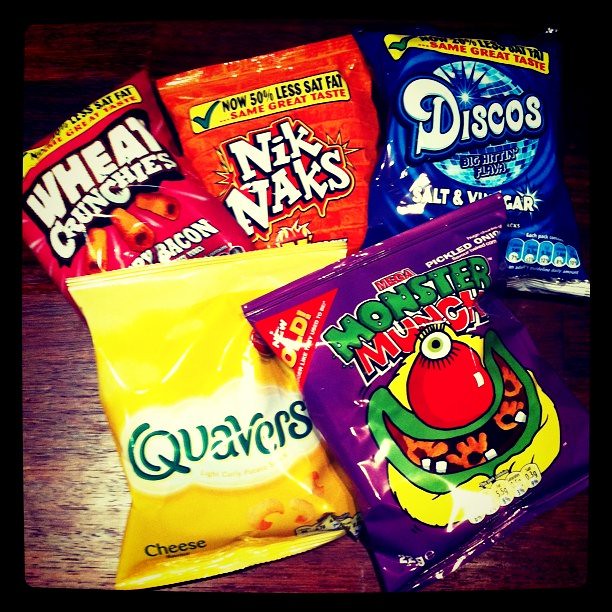This detailed photograph showcases a vibrant assortment of five snack packages laid out on a dark wooden table, all framed within a black, nearly square border. The arrangement features three snack bags on top and two on the bottom. In the top row, the leftmost is a red bag of Wheat Crunchies, the center also holds a red bag of Knick Knacks, and the rightmost is a blue bag of Discos, flavored with salt and vinegar. In the bottom row, the left side has a yellow bag of Quavers, which contain cheese, and the right side displays a purple bag of Monster Munch, featuring a whimsical monster with a big nose, big mouth, and one eye. The vivid and playful packaging designs, accentuated by bright artificial lighting, make the snack bags appear highly colorful and attention-grabbing, reminiscent of children's snacks.